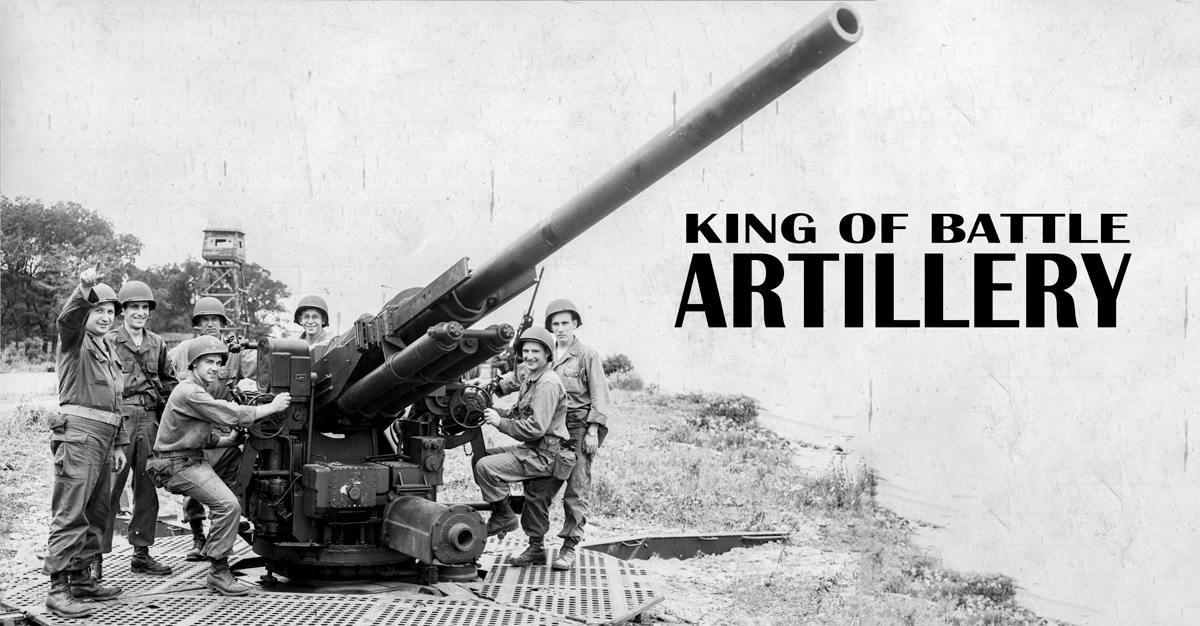In this striking black and white photograph from the World War II era, seven soldiers are gathered around a massive artillery cannon, positioned diagonally from the bottom left to the top right at a 30 to 40 degree angle. All are clad in period military uniforms, complete with protective helmets and fatigues, standing on a sturdy metal base. To the left of the cannon, five soldiers are positioned: the first stands with his right arm raised skyward, catching the viewer's eye; beside him, a smiling soldier stands closely, followed by a kneeling comrade who keeps one hand on the cannon. Behind them, another soldier stands unsmiling, while the final soldier in this group smiles gently. On the right side of the cannon, a soldier confidently holds a wheel—likely used to adjust the cannon's angle—with his foot braced on the metal base, smiling as well. Behind him stands another unsmiling soldier. All eyes are directed toward the camera, creating a sense of unity and purpose. The photograph is devoid of extensive scenery, emphasizing the men and their formidable weapon. Overlaid text reads "King of Battle Artillery," potentially signifying the unit's designation or motto.